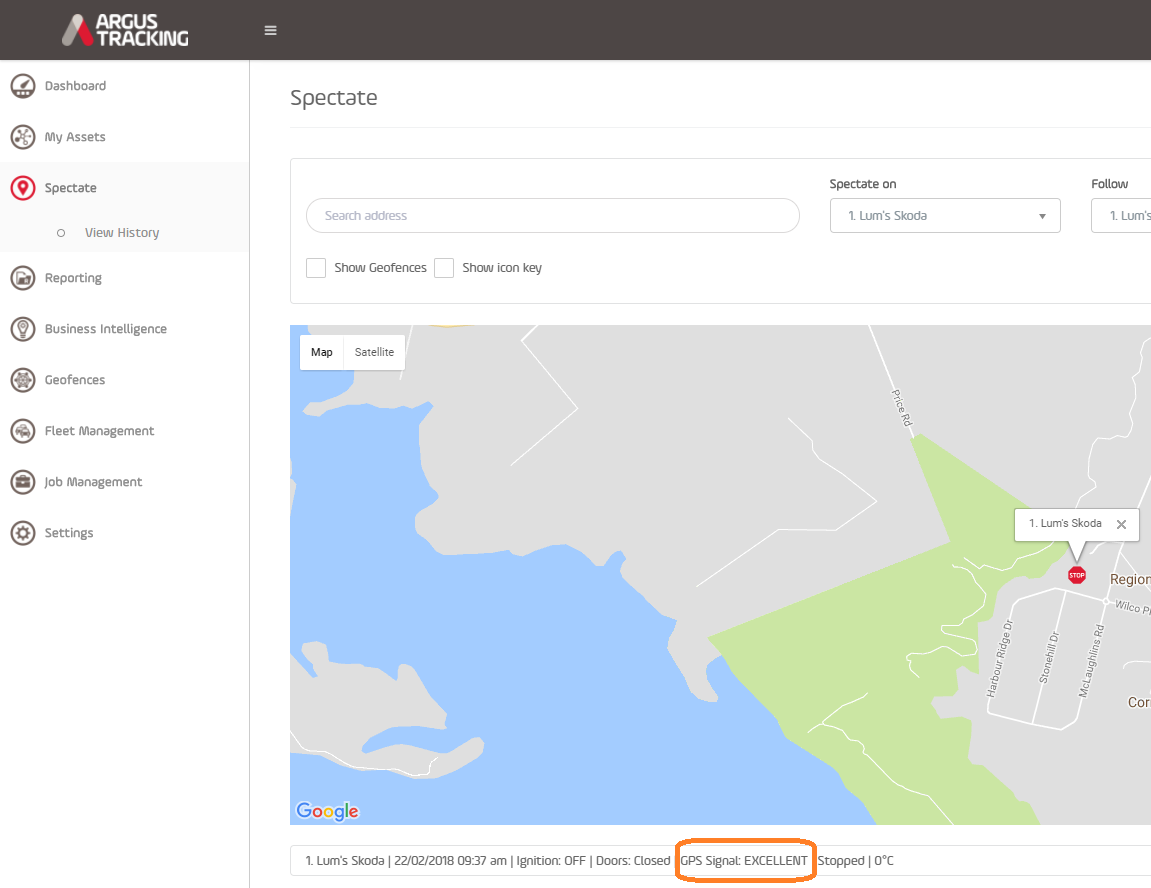This screenshot is from the Argus Tracking web application, specifically showcasing the 'Spectate' feature, which allows users to monitor the location of their assets. The layout includes the Argus Tracking logo positioned on the left side of the interface. Adjacent to the logo is a sidebar menu listing various options: Dashboard, My Assets, Spectate (which is currently selected), View History, Reporting, Business Intelligence, Geofences, Fleet Management, Job Management, and Settings. 

The central area of the screen displays a detailed map. Above the map, there are search and display options such as "Search for Address" and "Show Geofences." Users can also toggle the map view to Satellite mode. 

Currently, the map is pinpointing a location labeled as "Lums, Goda." Below the map, a GPS status section provides critical information: the date and time are February 22, 2018, at 9:37 AM. The ignition status of the tracked asset is off, the door status is closed, and the movement status indicates that the asset is stopped. The temperature is recorded at 0 degrees Celsius. Additionally, the GPS signal is shown to be excellent, highlighted with an orange outline. 

It appears that the person using this feature might be experiencing an issue, despite the excellent GPS signal strength, as they have possibly posted this image seeking assistance.